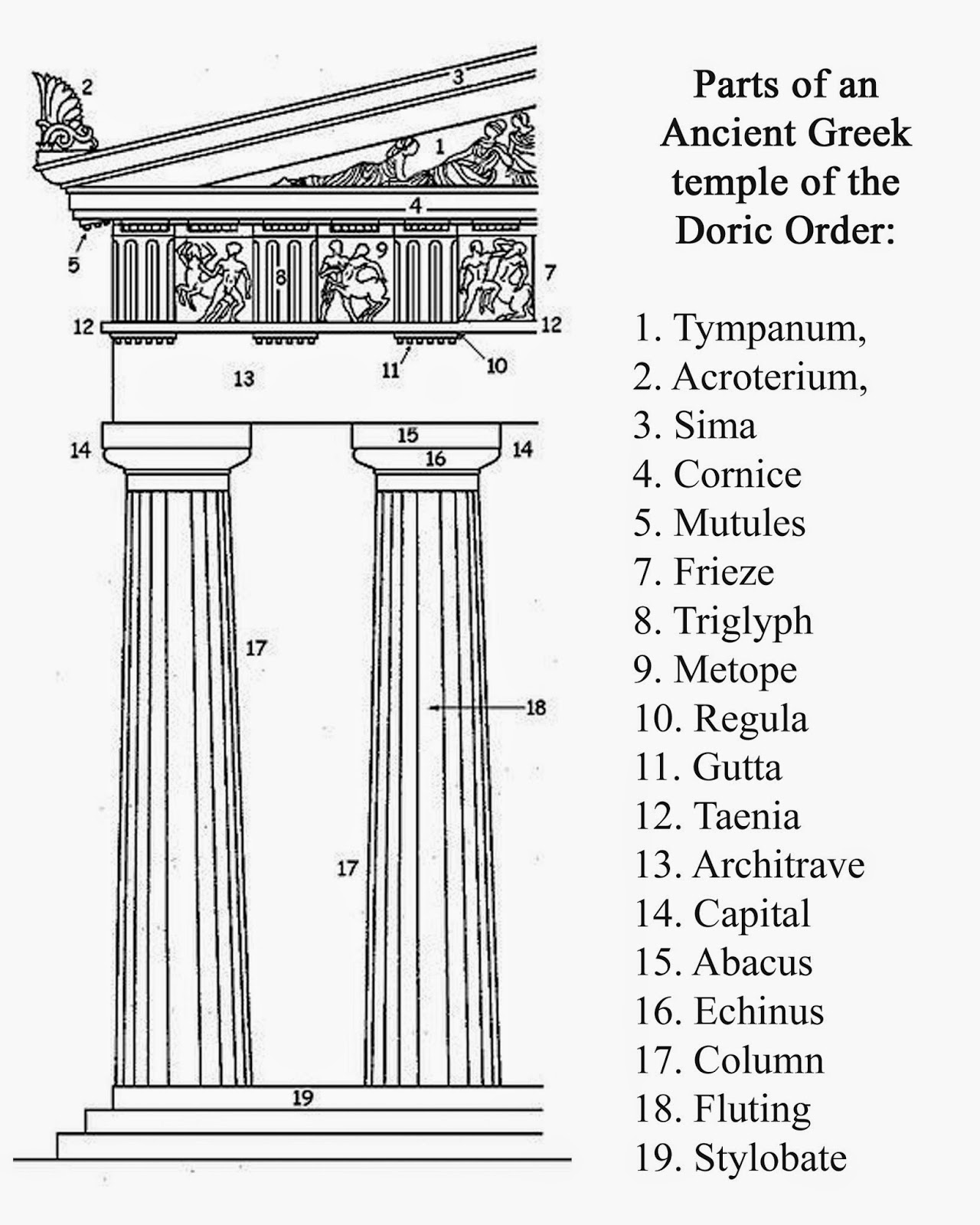The black and white image displays a detailed diagram of parts of an ancient Greek temple of the Doric order. On the left side of the image, there is a labeled drawing of the front side of the temple structure. At the top of the temple's front, there is a half triangle, known as the tympanum, adorned with a shell-shaped pattern at its tip. Below the tympanum, vertical line patterns are interspersed with a logo depicting human figures. Supporting this structure are two large pillars, standing in front of a flight of three stairs. Additional details include artistic depictions of women resting, a man riding a horse, and men engaged in combat. Each part of the temple is meticulously labeled, ranging from number one, the tympanum, to number nineteen, the stylobate. On the right side of the image, a title reads, "Parts of an Ancient Greek Temple of the Doric Order," with corresponding text and labels that match the numbered sections depicted on the left.